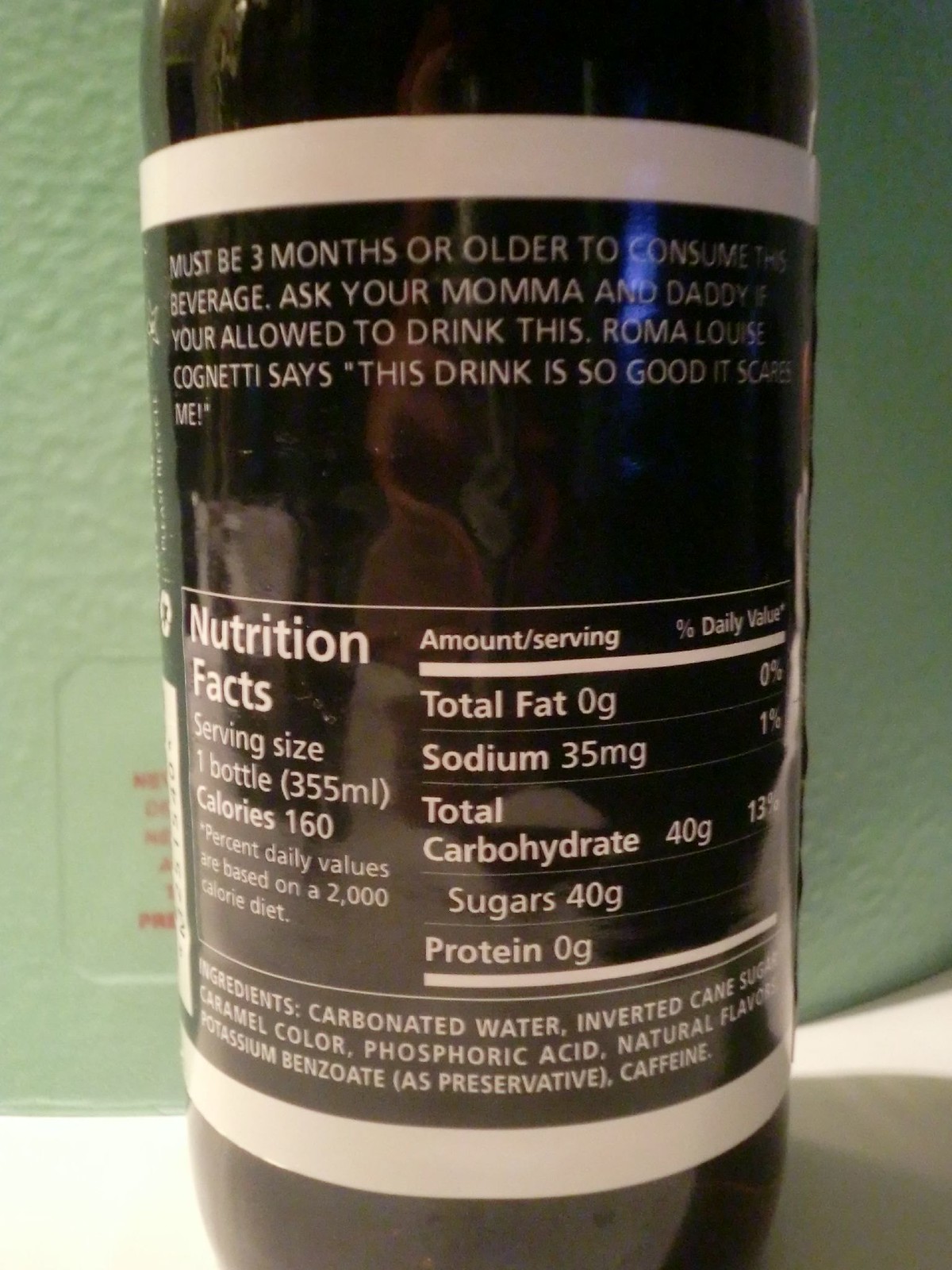A tightly cropped photograph showcases a dark brown, almost black bottle with a black-and-white label, prominently displaying its nutrition information. The bottle sits on a white surface, and the background reveals a textured wall with an indistinct label partially visible behind the bottle. 

At the top of the bottle's label, there is white text that reads, "Must be three months or older to consume this beverage. Ask your mama and daddy if you’re allowed to drink this." Below this, the label bears a whimsical endorsement, "Roma Louise con Yeti says this drink is so good it scares me."

Further down, the detailed nutrition facts are listed, including calories, fat, sodium, carbohydrates, sugars, and protein. At the very bottom of the label, the ingredients are outlined, with entries such as carbonated water, inverted cane sugar, caramel color, phosphoric acid, several longer chemical names, and caffeine.